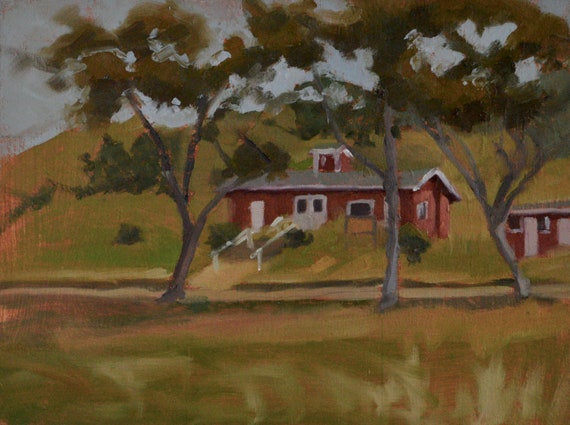This painting, created with traditional paints and brush techniques, showcases a charming single-story red house reminiscent of a ranch-style home. The focal point of the house is the pristine white front door, accessible via a ramp. A prominent chimney adds character to the structure. Several windows punctuate the façade, offering a glimpse into the cozy interior. Adjacent to the house stands a smaller red structure, possibly a barn or a playhouse, adding to the rural ambiance. 

The scene is framed by large, verdant trees, their leaves rendered in various shades of green to capture the play of light and shadow. The house is bordered by a dirt road or driveway, which meanders through patches of grass, suggesting a rustic, countryside setting. In the background, gentle hills complete the picturesque landscape, while a sky filled with soft, billowing clouds provides a serene backdrop. The entire composition is meticulously detailed, capturing the beauty and tranquility of a rural homestead.